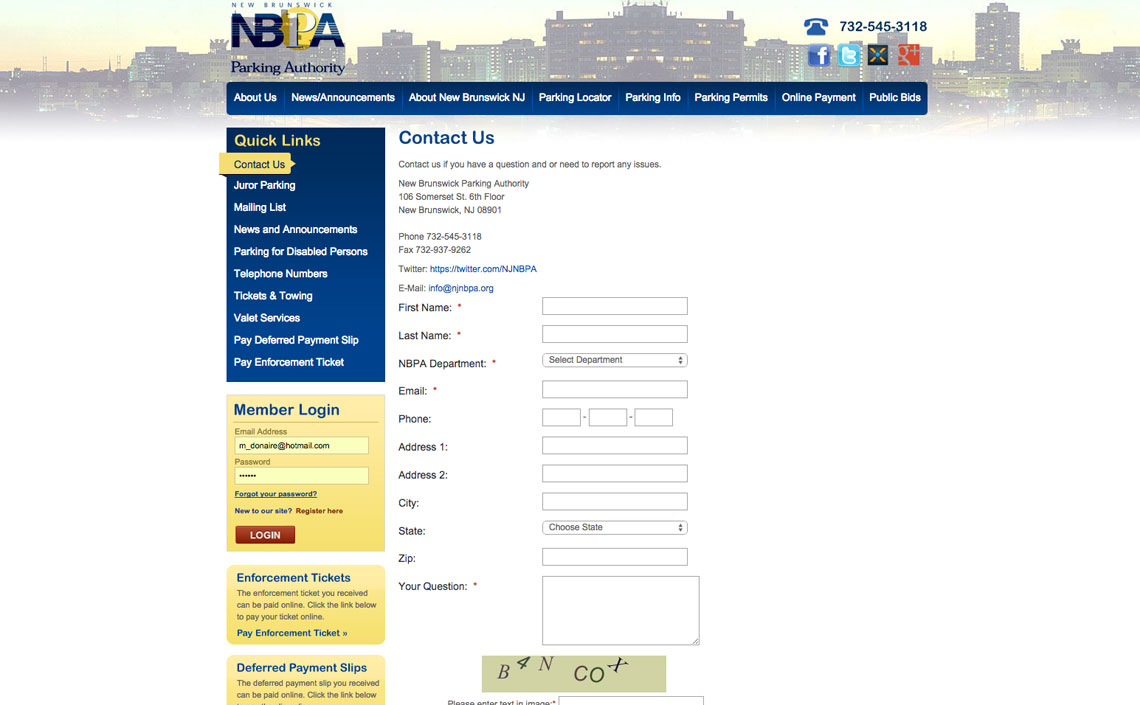This image appears to be a screenshot of a webpage from the New Brunswick Parking Authority (NBPA). The faded background prominently features an illuminated cityscape of New Brunswick, New Jersey, creating a visually engaging backdrop. The navigation menu at the top includes options such as "About Us," "News Announcements," "About New Brunswick, New Jersey," "Parking Locator," "Parking Info," "Parking Permits," "Online Payment," and "Public Bids."

Highlighted in the menu is "Contact Us," which provides information for inquiries or issues. The address is listed as New Brunswick Parking Authority, 106 Somerset Street, 6th Floor, New Brunswick, New Jersey, 08901. Additional services and information available include "Juror Parking," "Mailing List," "News and Announcements," "Parking for Disabled Persons," "Telephone Numbers," "Tickets and Testing," "Towing," "Valet Services," "Paid Deferred Payment Slip," and "Pay Enforcement Ticket."